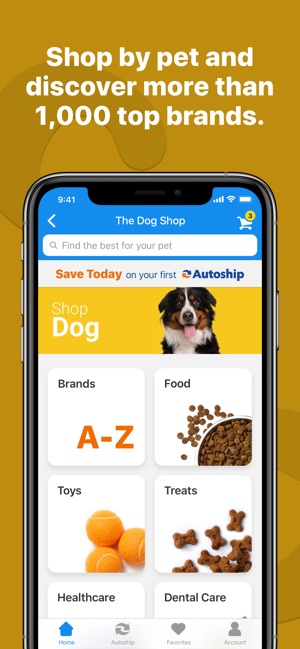Promotional Image for Pet Shopping Application

In this brightly colored advertisement, a vibrant yellow and dark yellow background highlights the promotion of a pet shopping application. The central message, "Shop by pet and discover more than a thousand top pet brands," invites users to explore an extensive selection of pet products.

A smartphone displaying the app screen is prominently featured, with the app interface showcasing "The Dog Shop." The phone screen also includes standard interface elements like the carrier signal, Wi-Fi signal, and battery life indicators, all set against a blue background. A white cart icon with an orange number "3" signifies an active shopping cart, suggesting three items already added.

At the top of the smartphone screen, a Border Collie is pictured, contextualizing "The Dog Shop" theme. Below, a bright orange section of the screen promotes a special offer: "Save today on your first auto-ship." 

The app's interface appears user-friendly, with options such as "Brands A to Z," "Food," "Toys," and "Treats" prominently displayed. Icons next to each category illustrate the type of products: tennis balls for toys and pet treats for treats. The food category shows a food dish filled to the brim, while additional options for "Health Care" and "Dental Care" complete the comprehensive list of offerings.

Overall, the advertisement effectively communicates the diverse range of products available through the app, enticing pet owners with the promise of convenience and variety.